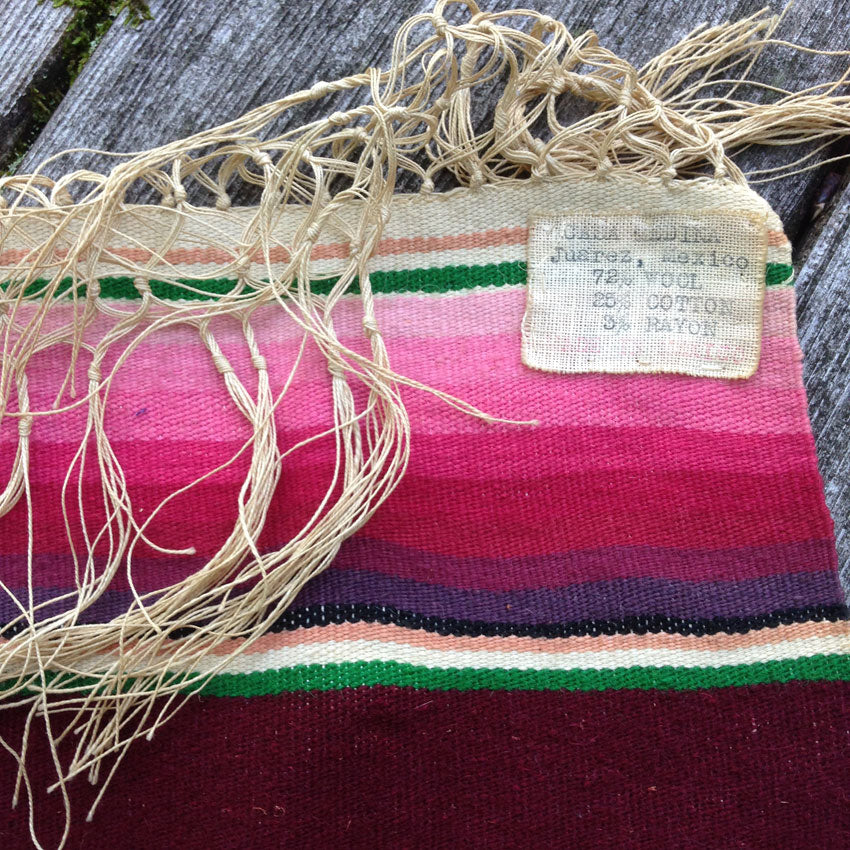This image captures a vibrant and intricately woven Mexican blanket adorned with tassels. The blanket is draped over an old, weathered wooden surface, which adds a rustic charm to the scene. The blanket's pattern unfolds in a harmonious gradient of colors starting with soft tan tassels that lead into a tan stripe, followed by a thinner brown band. It transitions through a sequence of thin stripes ranging from green, light pink, and progressively darker pinks into red shades. From there, it shifts to lavender and dark purple, continues with a bold black stripe, and finally concludes with a series of salmon, white, and green stripes. In the upper right corner of the blanket, there is a small, slightly worn product label from Juarez, Mexico, indicating the composition of 72% wool, 25% cotton, and 3% rayon.